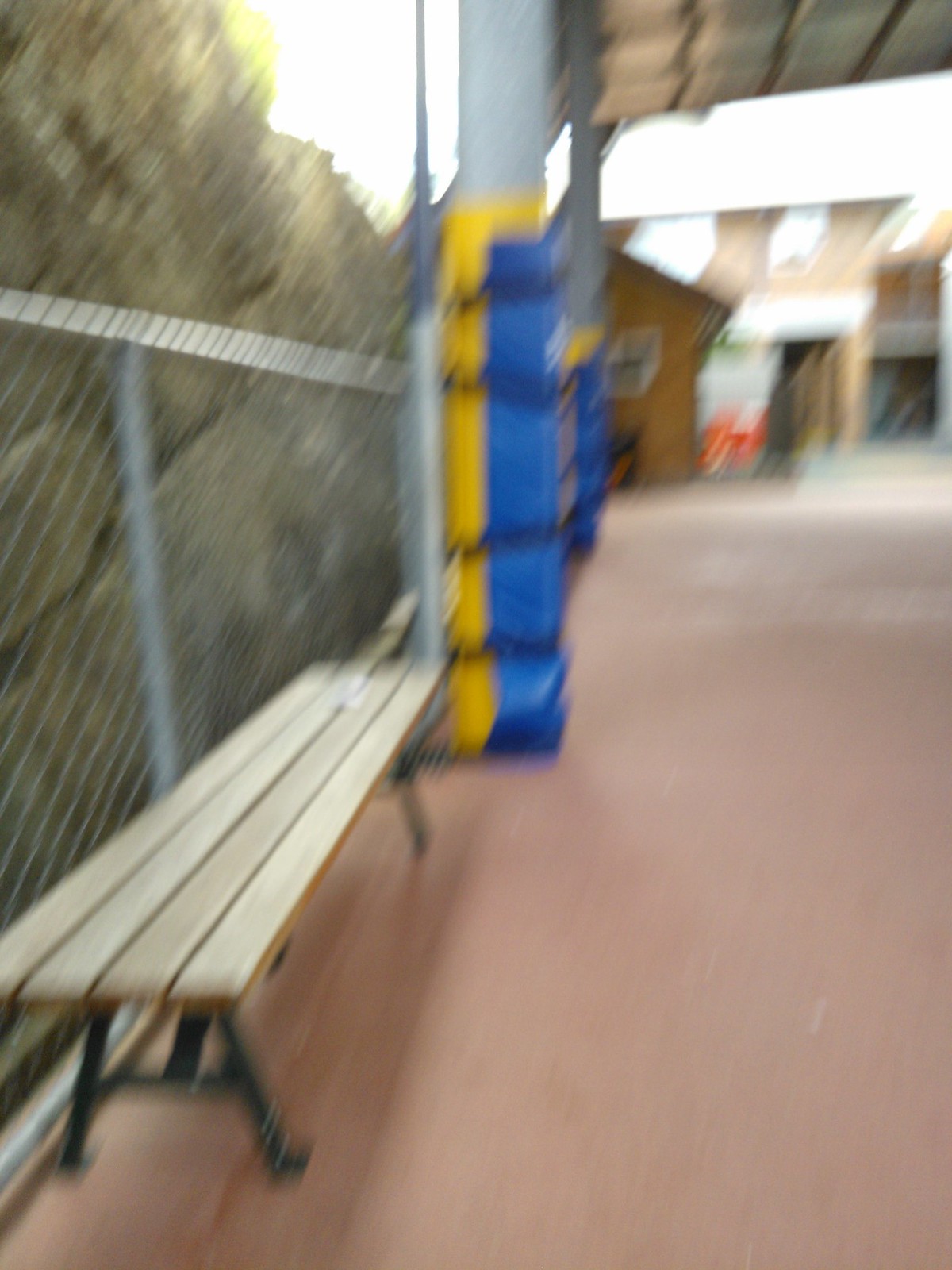The image depicts an outdoor scene captured in bright sunlight, though it is significantly blurry and grainy. Dominating the foreground is a backless wooden bench with metal legs, positioned in front of a chain-link fence. The fence stands against a tall rock formation that gives a rugged, natural backdrop to the scene. 

To the right of the bench, extending away from the viewer, there are two gray pillars wrapped with blue and yellow padding, likely for safety purposes. Farther back, blurred buildings can be seen; the one closest to the bench appears to be a single-story structure, possibly wooden, with a dark window framed in white. To the right of this building, there is a tan, possibly two-story building with multiple windows and a roof that blends into the bright sky, obscured by overexposure. The overall atmosphere suggests an outdoor recreational or public space, with multiple elements blending into a slightly chaotic yet intriguing visual.